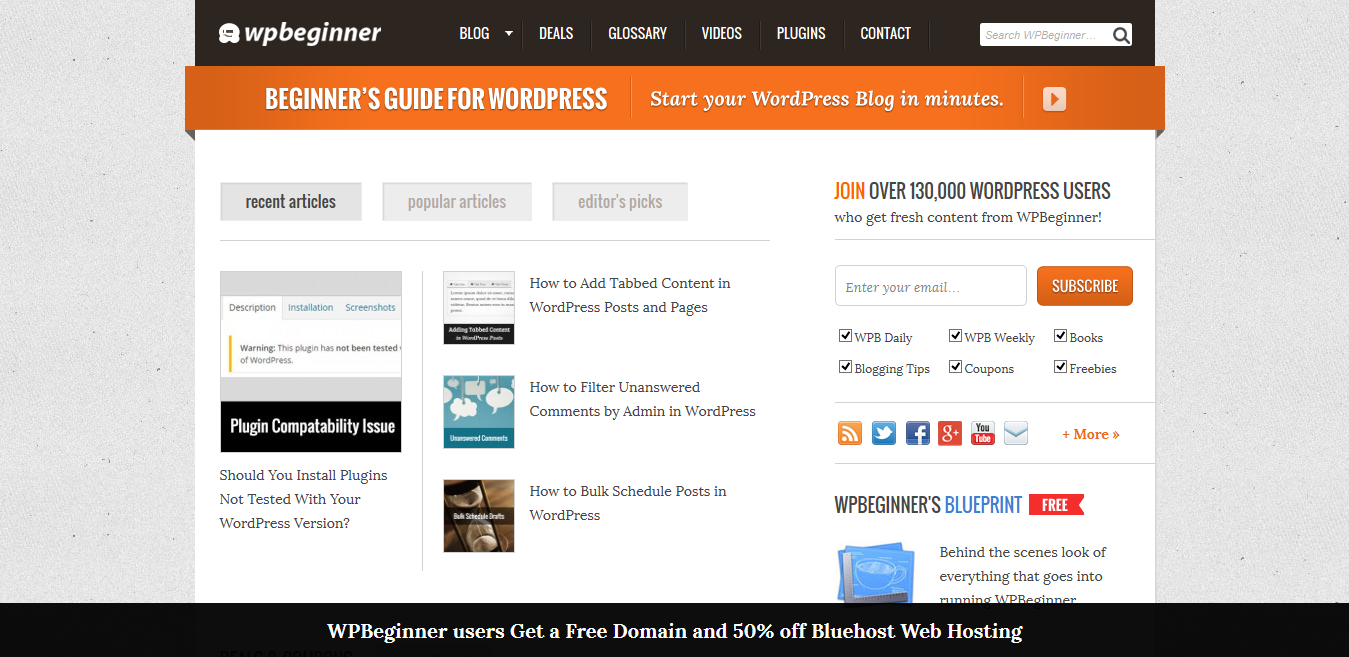#### Detailed Caption:

This is a screenshot of a web page from WPBeginner, featuring a detailed layout and various sections relevant to WordPress users. 

At the top, bordered by a black bezel, the left-hand side features a distinctive white circle containing smaller white circles with the letters "WP" prominently displayed. This represents the WPBeginner logo.

Below the logo, there is a navigational menu with clickable sections, all written in white uppercase text, ordering as follows: BLOG (with a down arrow indicating a dropdown menu), DETAILS, GLOSSARY, VIDEOS, PLUGINS, CONTACT. Adjacent to this menu is a white rectangular search bar bordered with gray, featuring the text "Search WPBeginner" beside a black magnifying glass icon.

Beneath the navigation menu, there is an orange rectangle with bold white text that reads, "Beginner’s Guide for WordPress." To the right of this, in italicized text, it says, "Start Your WordPress Blog in Minutes." 

Adjacent to these informational blocks, there is another orange square containing an overturned gray triangle on its right-hand edge. Below this section, several dark gray rectangular buttons offer more content, reading: RECENT ARTICLES (in black text), POPULAR ARTICLES (in gray), and EDITOR'S PICKS (also in gray).

On the left-hand side of the screenshot, there is a portion of another web page with a light gray background displaying multiple tabs. The selected tab is highlighted in white with black text that says "DESCRIPTION," followed by an orange line and bold black text reading "WARNING." The subtext underneath reads, "This plugin has been tested…" but is cut off, pertaining to WordPress plugin testing. Additional tabs, "INSTALLATION" and "SCREENSHOTS," are shown in mid-gray with hyperlink blue text.

In the dark black bezel below these tabs, bold white text reads, "PLUGIN COMPATIBILITY ISSUE." Accompanied by regular black text, it poses the question, "Should you install plugins not tested with your WordPress version?"

Additional sections on the web page feature various tips and guides with corresponding graphics. A detail reads, "How to add tabbed content in WordPress posts and pages," positioned adjacent to a gray and black webpage image. A cyan blue square with dark blue bottom accents displays circles and rectangles representing interface elements, with the guide "How to filter unanswered comments by admin in WordPress" in gray text on the right.

Another webpage detail shows a black hourglass with white sand on a wooden surface, captioned "How to bulk schedule posts in WordPress."

Finally, on the right-hand side, an invitation in bold orange and black text reads, "Join over 130,000 WordPress users who get fresh content from WPBeginner!"